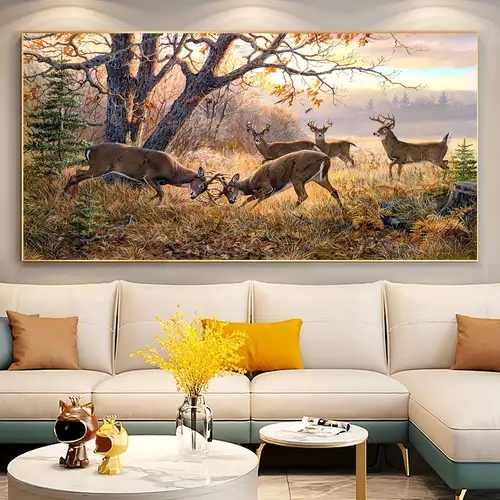In an elegantly furnished living room, a green and cream leather sectional sofa adorned with green, brown, and gold pillows sits beneath a large, horizontal painting. The painting, framed in thin gold, depicts a serene autumn scene with five deer; two of the deer are locking antlers while the other three look on amidst a landscape of green and tan ground, brown grasses, and an oak tree shedding its orange leaves against a backdrop of blue skies, distant mountains, and soft cloud cover. In front of the sofa lies a white marble coffee table with golden legs, featuring two small cat statues—one brown and one yellow—alongside a clear glass vase holding vibrant yellow goldenrod flowers. The floor underneath is a light gray and tan marble slate, completing the cohesive décor of the room. Above the painting, three lights cast a gentle glow, highlighting the intricate details of the artwork and the inviting ambiance of the space.